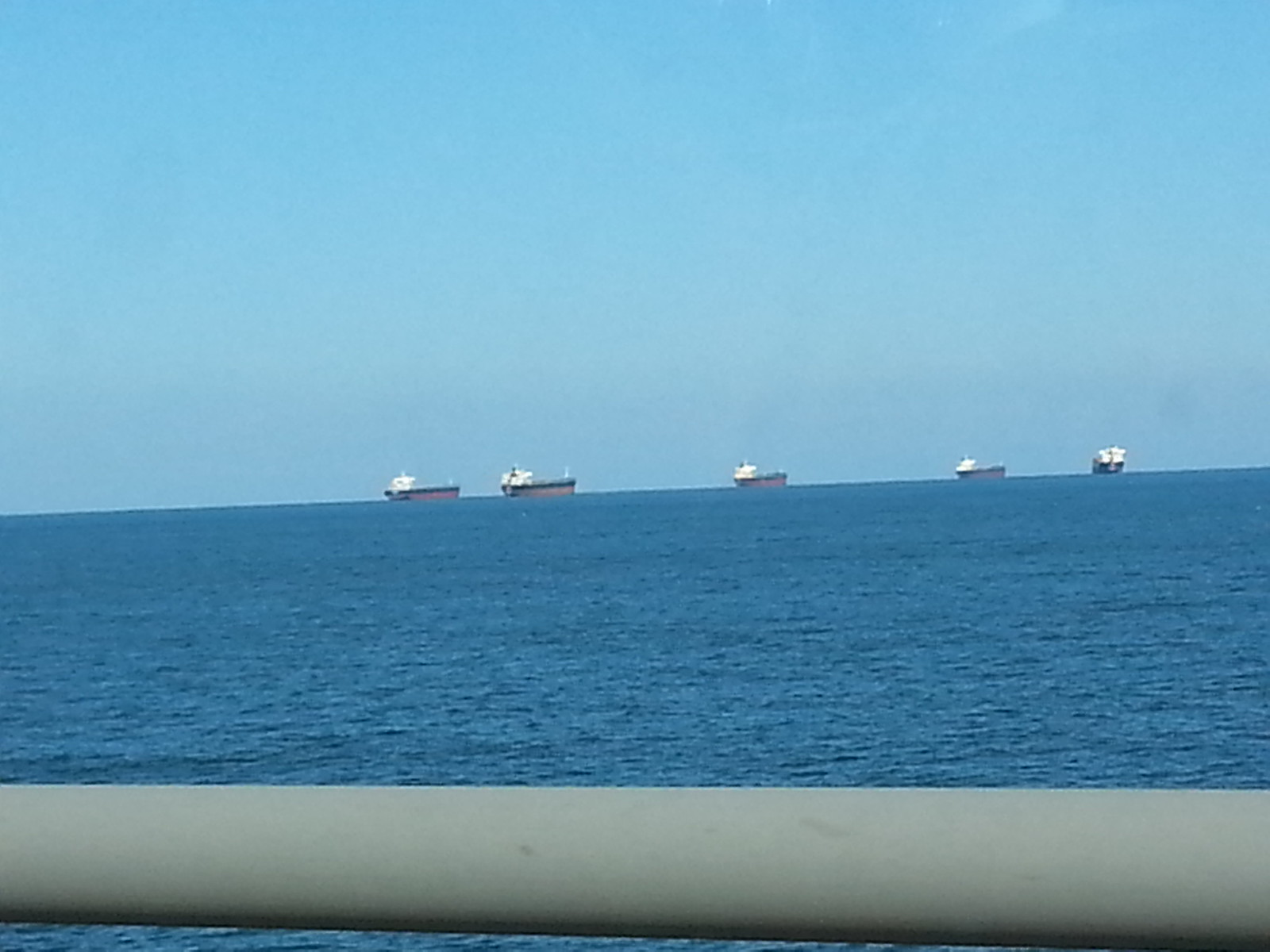The image captures a fleet of five large ships floating on the horizon of a vast, deep blue ocean. The photograph is taken from what seems to be another vessel, indicated by the presence of a smooth, grayish, round metal railing at the bottom of the image. This railing runs horizontally from left to right. About 30% of the image is dominated by the ocean's expanse, transitioning into the horizon line where the five ships are visible. The sky above is a clear, cloudless blue, enhancing the serene and expansive maritime scene.

The ships, likely tankers or container ships, are characterized by their distinct color patterns: the bottom sections that are barely above the waterline are painted red, followed by a black stripe, and topped with a white superstructure. Four of these ships are oriented side-on to the viewer, while one on the far right appears to be facing forward, adding a subtle variation to the composition. The overall scene is tranquil, with a uniform sky meeting the calm expanse of the ocean at the horizon, dotted by these large vessels.